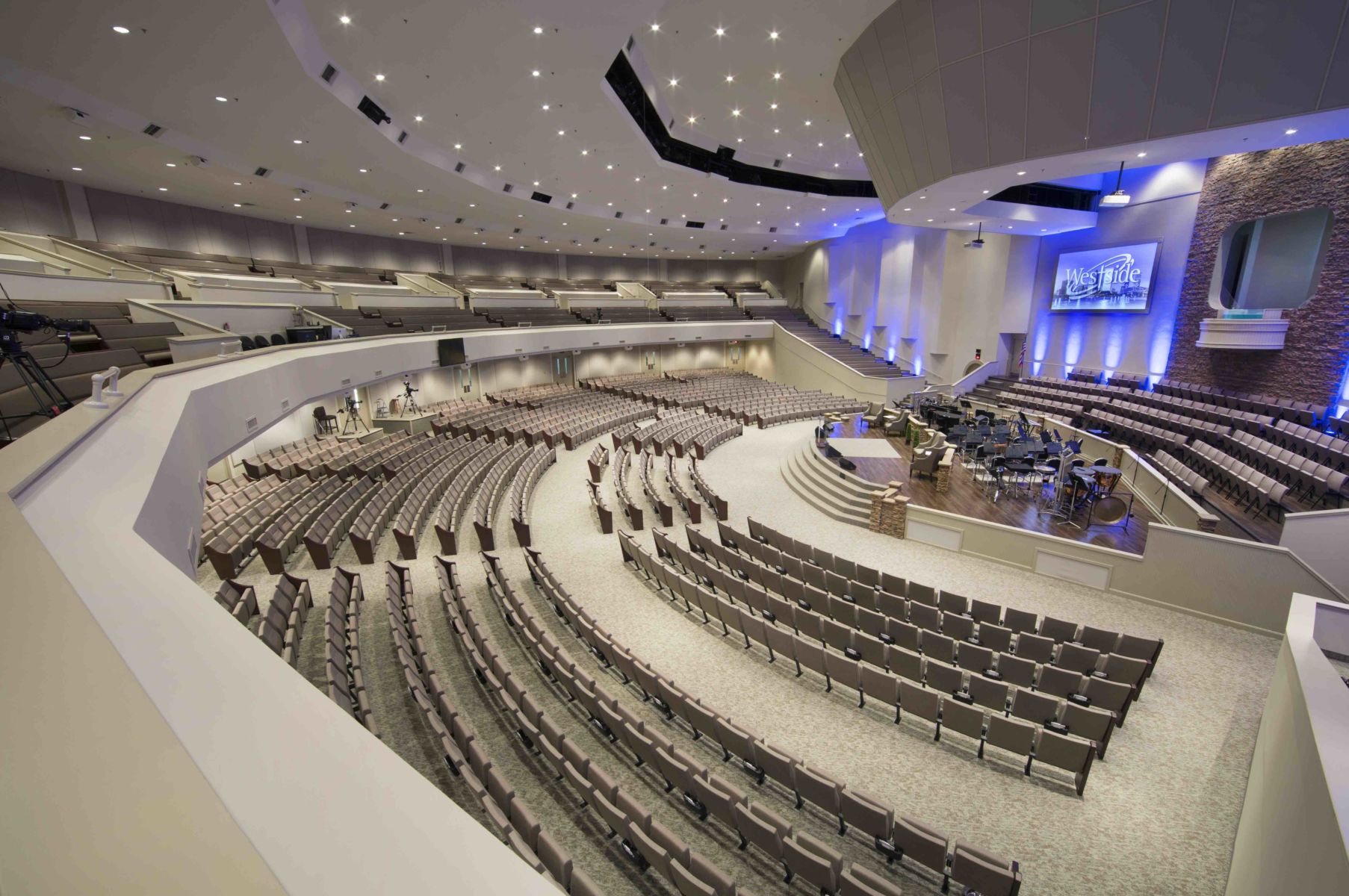The image depicts a large, modern venue that could serve as a theater, concert hall, or church. This spacious auditorium features neutral colors with beige, grey, and white dominating the scheme. The seating is arranged in a semi-circle on the ground floor and continues into a mezzanine or balcony level, ensuring good visibility from all areas. The ground floor has multiple rows of light grey, liftable seats, while the mezzanine has white walls and is separated by a simple wall divider. At the back of the ground floor, cameras can be seen, suggesting events here are recorded.

The centerpiece of the venue is a prominent stage with a wooden floor adorned with chairs, resembling a setup for a talk show or an orchestra. The stage also houses some musical instruments, including a drum set. Behind the stage, there are more chairs arranged, likely for a choir. A significant digital or plasma screen displays the words "West Side" encircled in white, which could be a logo or name associated with the venue. Additionally, there are spotlights and lighting effects from the white ceiling, contributing to the modern and well-lit atmosphere of the hall. The overall capacity of the venue suggests it can accommodate hundreds of attendees, making it suitable for a variety of large-scale events.